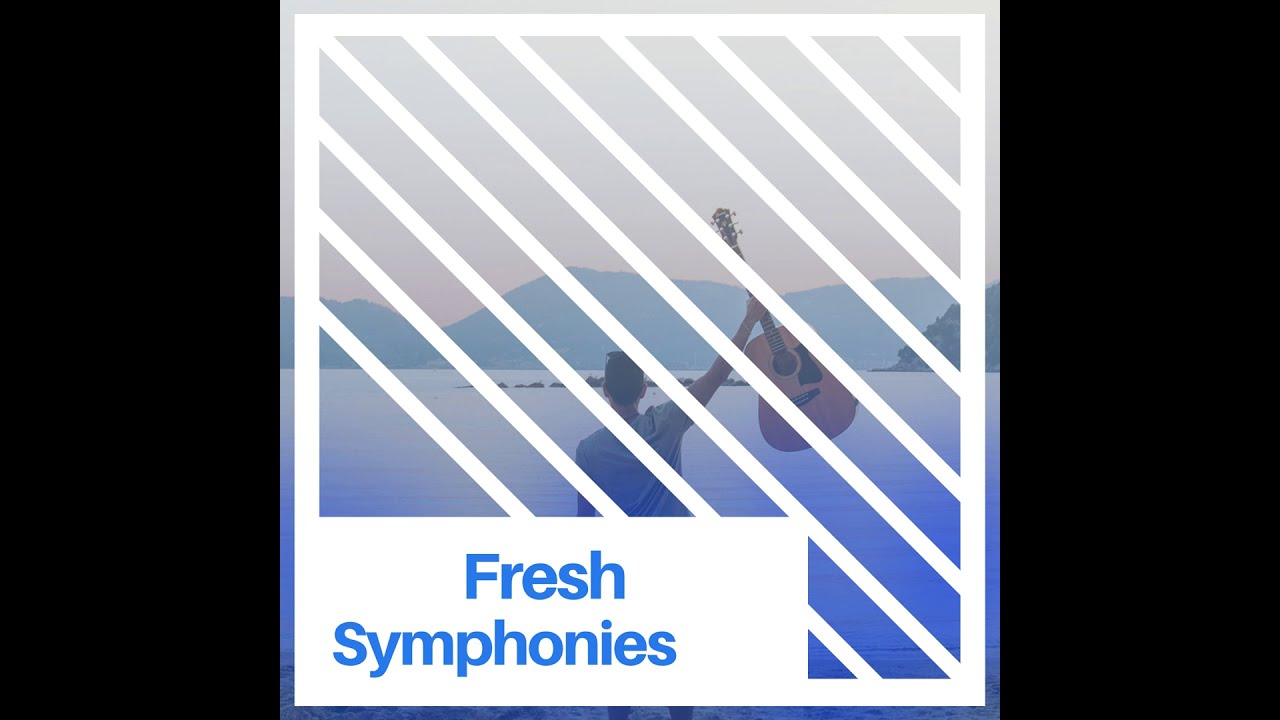The image showcases a CD album cover featuring a central square photo set against a black background, with black borders on the left and right sides. Diagonal white lines traverse the square image, partially obscuring a man who stands with his back to the viewer, raising an acoustic guitar in his right hand. The setting is outdoors, framed by a large body of water that transitions from light blue to a deeper violet hue, with distant mountains silhouetted against a gray sky. On the bottom left of the square, a rectangular white section contains the text "fresh symphonies" in blue. The cover captures a serene yet dynamic scene, reflecting both natural beauty and musical elements.